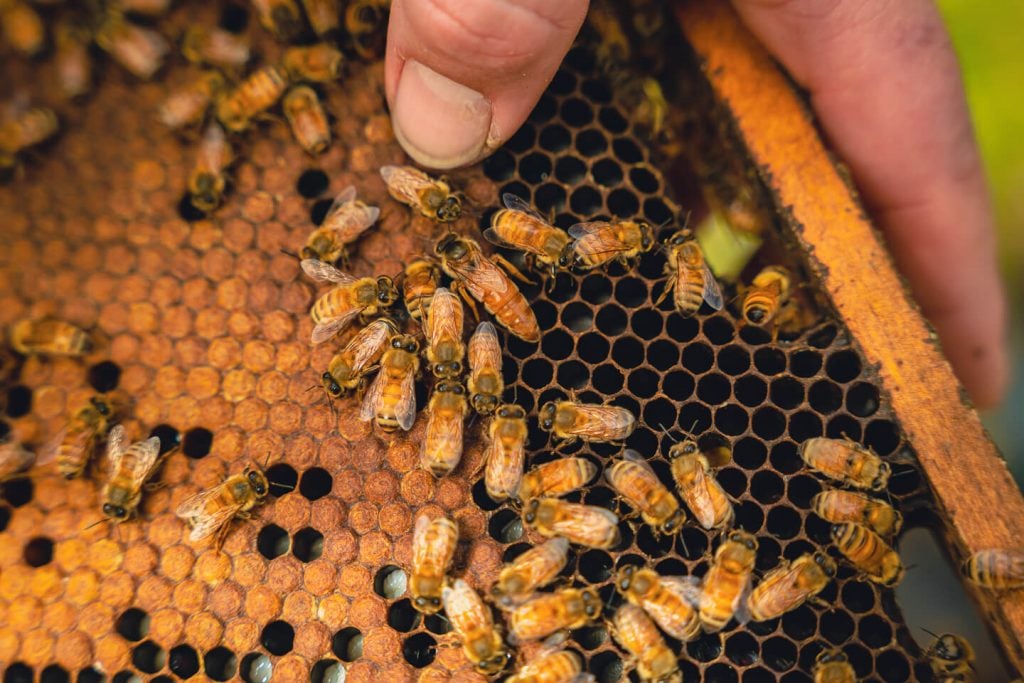This detailed close-up photograph captures a beekeeping frame being held by a man's hand. The frame, made of golden brown wood, shows some deterioration on the right edge. The man's thumb is prominently in focus, revealing a callus and dirt under his fingernail, while his finger is slightly blurred. The honeycomb panel on the left side is filled and covered with a brown texture, whereas the right side reveals empty honeycomb cells. Approximately 25 to 30 bees are seen actively moving across the frame, with some flying. The queen bee is central among the bees, surrounded by attentive worker bees. In the background, there is a hint of grass, but the main focus remains on the bees and honeycomb. The photo is color, with no text or additional objects, emphasizing the intricate details of beekeeping.